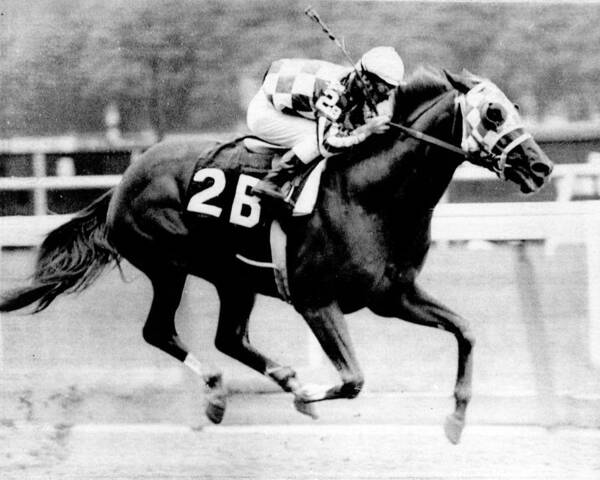This vintage black-and-white photograph captures a dramatic moment during a horse race. The dark-colored racehorse, numbered 2B, is captured mid-gallop with all four legs off the ground, illustrating its impressive speed on what appears to be a dirt track. The horse is equipped with the essentials: a saddle and a bridle. The jockey, in a streamlined, aerodynamic position, is clad in a distinctive uniform comprising light-colored pants, a dark-and-light checkered shirt, and a white helmet. The jockey grips both the reins and a riding crop, focused intently on the race. The background reveals elements of the racetrack, including the inner rail visible near the horse and farther off in the distance, with structures such as walls or fences lining the track. The motion blur in the background, along with the slightly worn quality of the image, emphasizes the speed and fervor of the moment while hinting at the presence of an audience watching this intense race unfold.